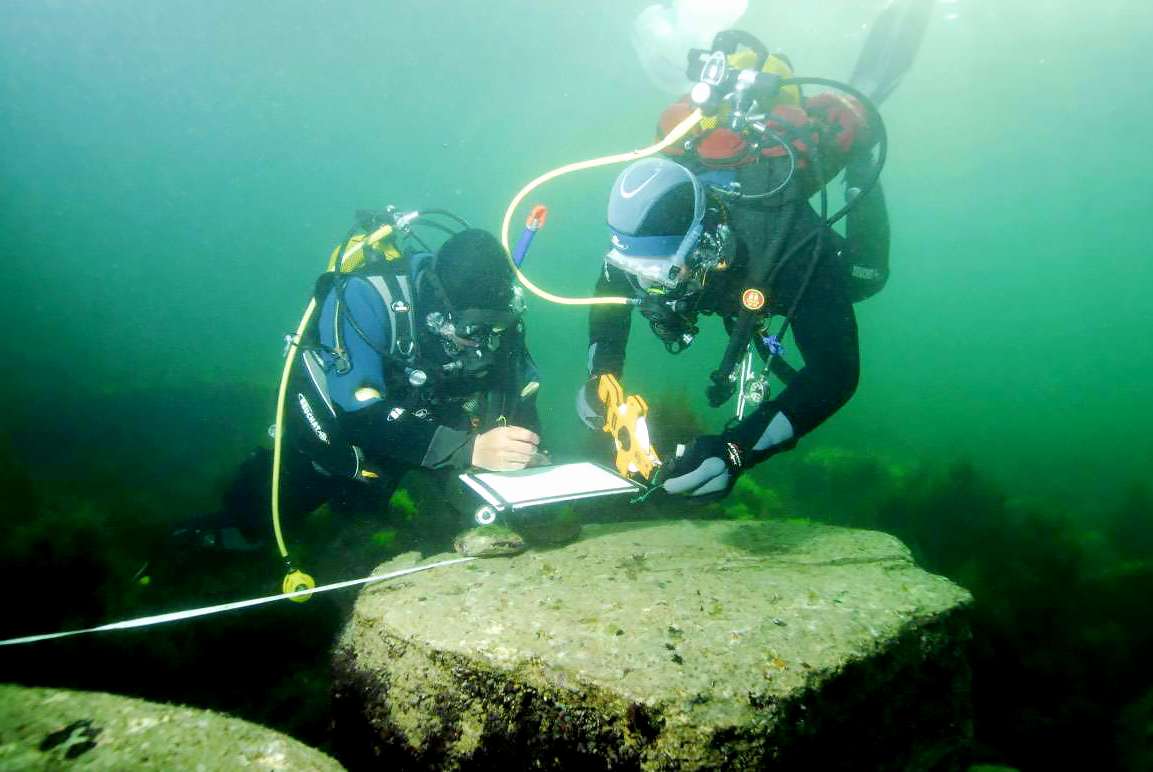The underwater photograph captures two scuba divers intently working above a large, flat, concrete structure, potentially an artificial reef. The divers, clad in well-fitted blue wetsuits, flippers, and equipped with breathing apparatus connected by air hoses, are submerged in a murky, bluish-green oceanic environment. The diver on the right can be seen with their fins trailing behind, while the diver on the left appears more grounded with feet planted on the seafloor. They are engaging with what seems to be a waterproof tablet resting on the concrete slab; one diver uses a stylus to write on the tablet, while the other holds a surveyor's measuring tape, possibly recording or measuring data. Their surroundings include patches of green seaweed scattered across the seabed. The divers' gear includes backpacks with tanks, though one tank might have a red marking, and the diver on the right is wearing gloves. The water around them is somewhat grainy, transitioning from a murkier blue at the top to a darker green toward the bottom.